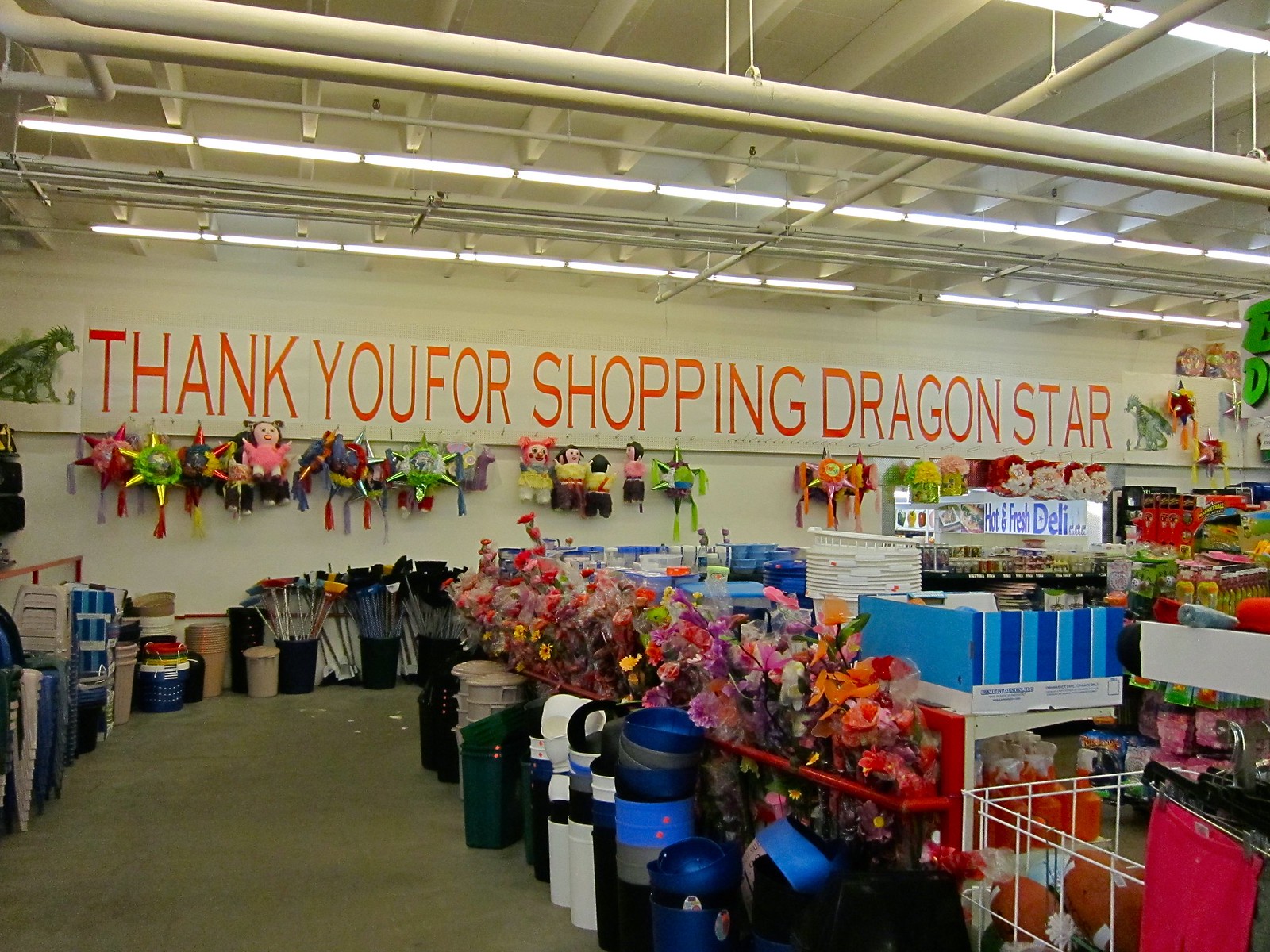The photograph is a vibrant and detailed depiction of the interior of a store. In the background, a brownish-beige wall prominently features an orange "THANK YOU FOR SHOPPING DRAGONSTAR" sign in capital letters, exuding a welcoming and thankful vibe. Overhead, the store has an industrial loft ceiling with exposed electrical and plumbing systems, interspersed with several hanging rod fixtures and small halogen lights illuminating the space.

To the right of the frame, a sign reads "HOT AND FRESH DELI," hinting at the presence of a prepared food section. The front area of the store captures a burst of colors and textures, displaying an assortment of fresh flowers, some wrapped in cellophane, with hues ranging from vibrant orange and gold to lush green.

Additionally, a chaotic yet intriguing collection of variously sized garbage cans occupies another section at the front. These bins come in green, blue, and black, contributing to the eclectic range of items available in this versatile store. The image overall portrays a bustling retail environment catering to a variety of customer needs.